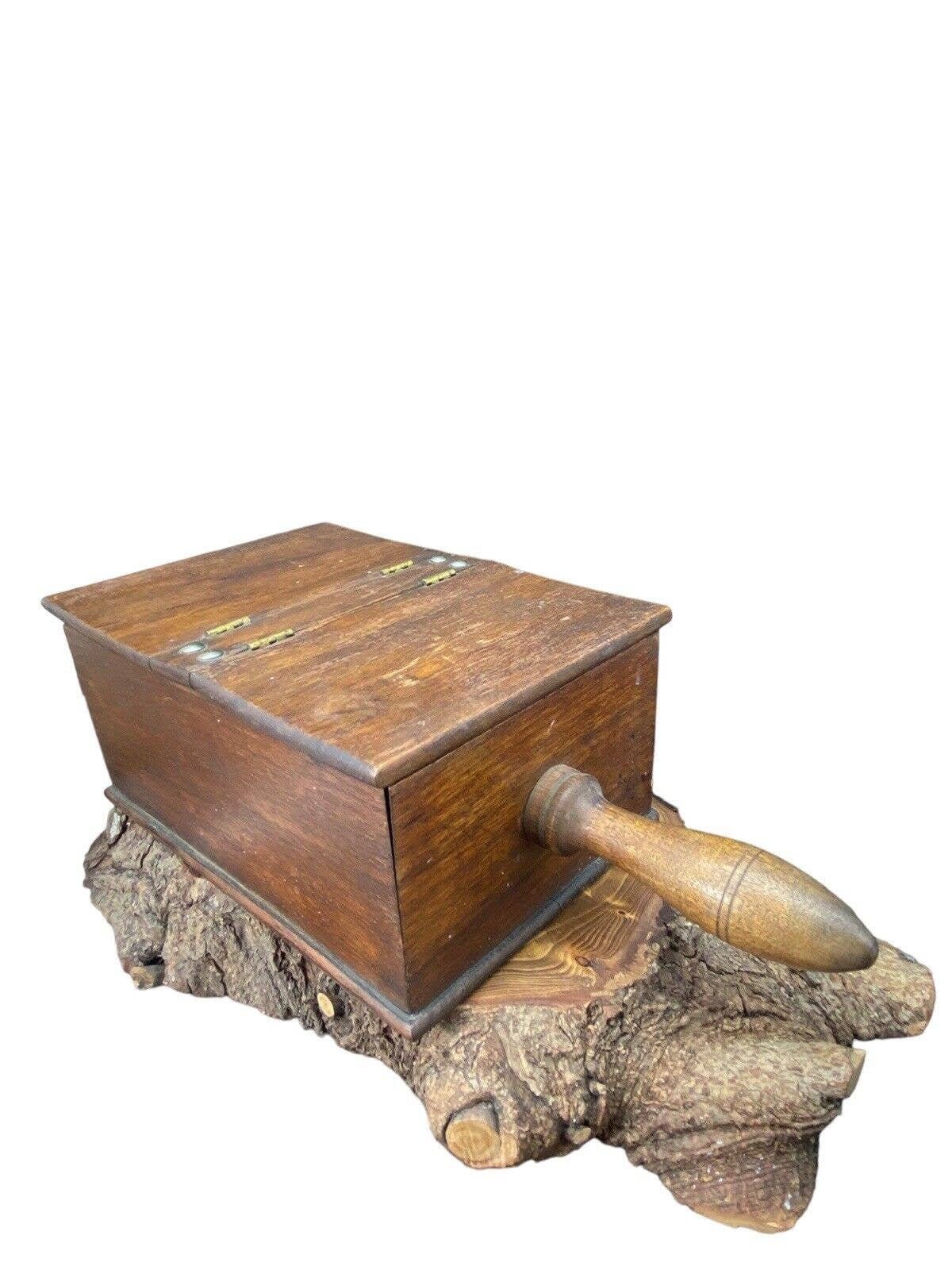This image depicts a close-up view of an antique, rectangular wooden box exhibiting significant signs of wear and age, such as scratches and a weathered surface. Crafted from a dark brown oak wood, the box features a large, prominent handle on its top, raising questions about its intended purpose. Hinges are visible along the top, indicating that both the front and back panels can be lifted upwards to open. The box's dimensions suggest it is relatively large and perhaps used for substantial storage. It is perched atop a thinly sliced tree stump, which serves as an elevated stand, with distinct patterns and rings visible on its grayish-brown surface. The setting of the image is against a plain white background, effectively isolating and highlighting the vintage box and its rustic stand.